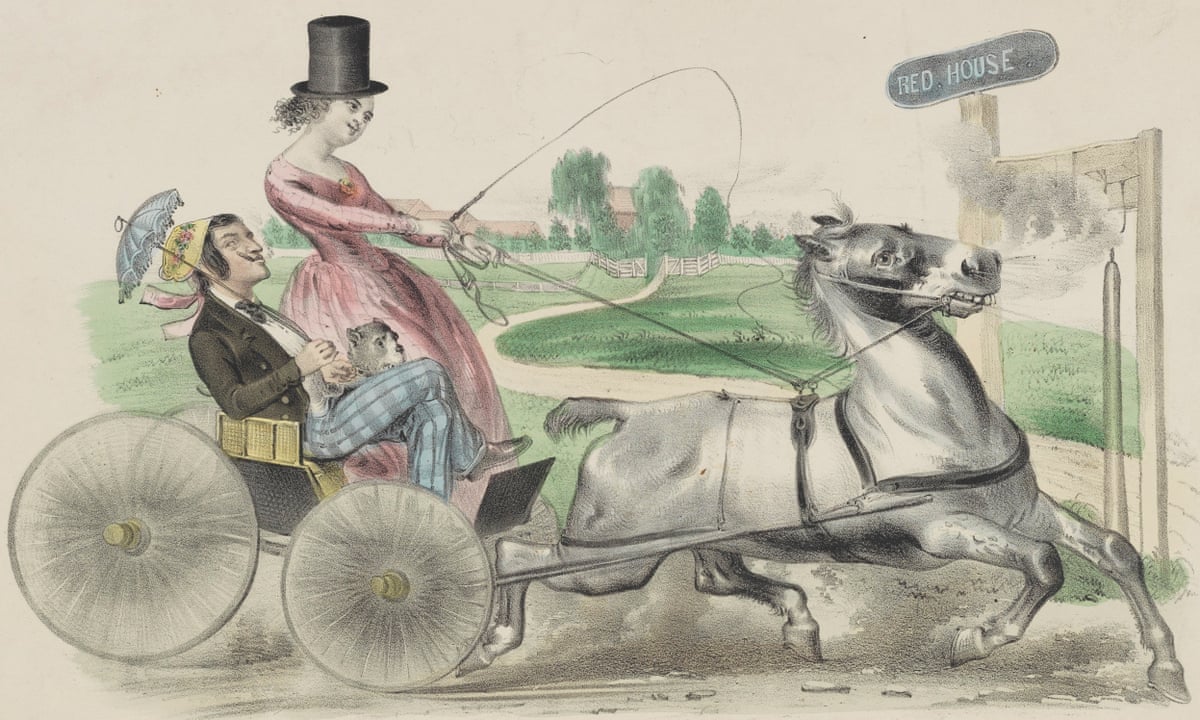The image is a detailed, colored drawing reminiscent of an early Victorian era illustration. It depicts an extraordinary scene with a man and a woman riding in a chariot-like cart, which has two wheels - the front smaller than the back. The man, wearing blue checkered pants, a black dress shirt, and a long-sleeved jacket, is oddly donning a bonnet and holding a small, light blue umbrella that matches the woman's parasol. He sits relaxed with his legs up, looking quite content, while a tiny, gray dog rests in his lap. The woman, dressed in a pink gown and a magician-style black top hat, appears exuberant as she commands the cart, holding the reins and a thin whip, urging their horse forward. The horse, a stout and visibly distressed gray stallion, seems out of place in its role, almost as if it can barely manage the task at hand. The backdrop features lush green trees and a winding road, placing the travelers in the midst of idyllic countryside scenery. A street sign labeled “Red House” suggests their destination, adding a touch of narrative to their whimsical adventure.